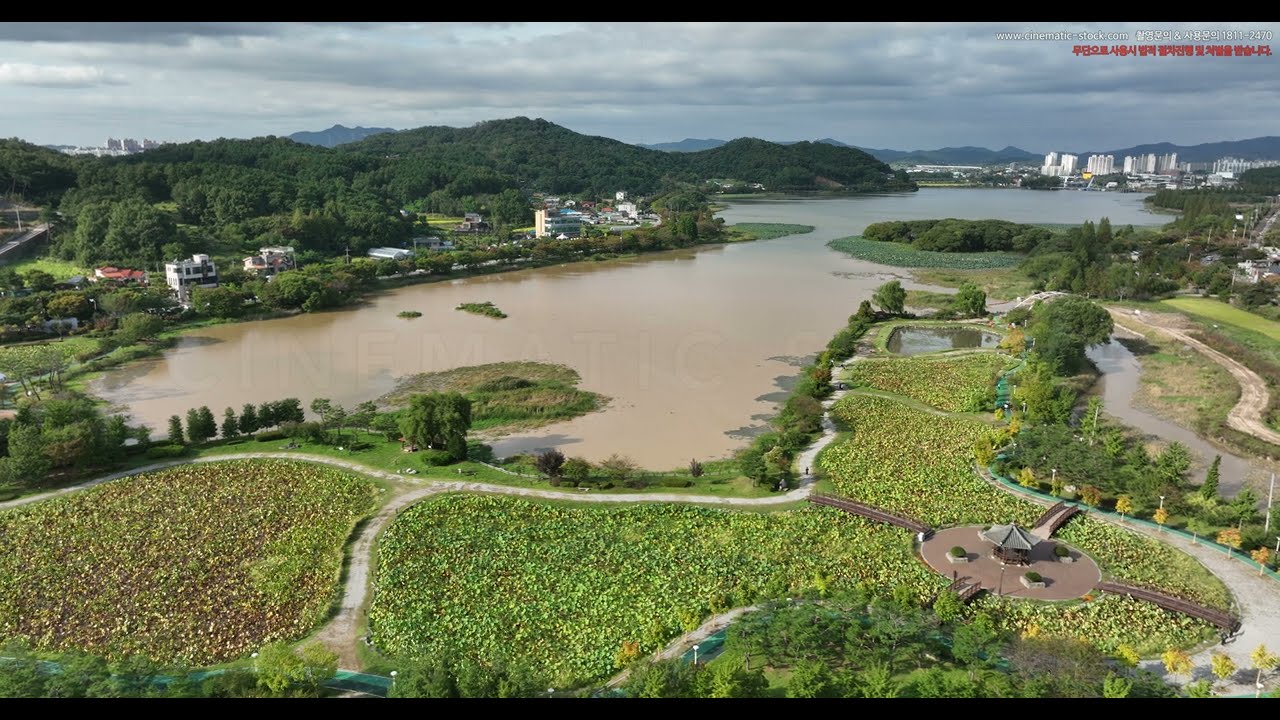The aerial image captures a scenic view of a large body of water, potentially a lake or inlet, characterized by its muddy, brown appearance. Surrounding the water, lush green grass covers the land, interspersed with winding gravel paths that thread through the verdant vegetation. To the right, a dense, wooded forest stretches toward distant mountains. Prominent in the image is a large gazebo with red brick flooring located in the bottom right corner, featuring a circular patio accessible by four gravel walkways extending in cardinal directions over a garden space. The backdrop reveals a sprawling cityscape with numerous towering skyscrapers clustered in the top right corner, while smaller office buildings, likely three or four stories tall, are nearer to the photo’s perspective. The scene appears partly cloudy, adding a serene ambiance to the picturesque setting.